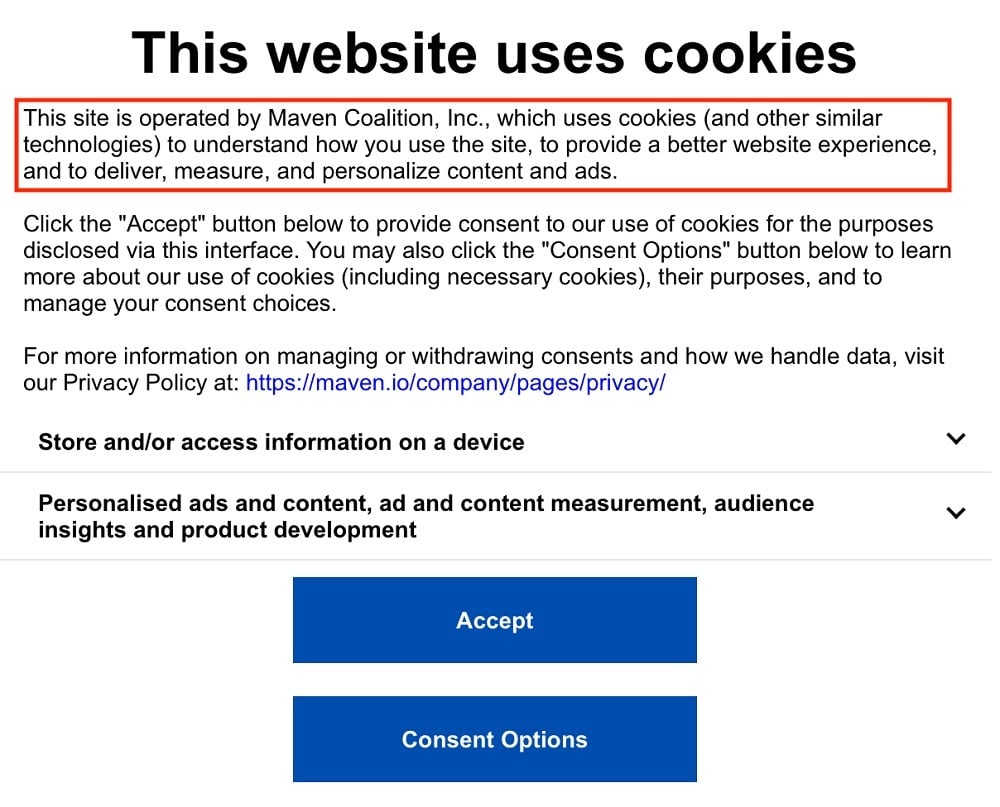The image displays a website's cookie consent agreement. At the top, prominent black text reads, "This website uses cookies." Below this, a red-bordered rectangle contains detailed information about the site's cookie usage. It states, "This site is operated by Maven Coalition Inc., which uses cookies and other similar technologies to understand how to use the site, to provide a better website experience, and to deliver, measure, and personalize content and ads."

Following this, the text instructs the user: "Click the 'Accept' button below to consent to our use of cookies for the purposes disclosed via the interface. You may also click the 'Consent Options' button below to learn more about our use of cookies, including necessary cookies, their purposes, and to manage your consent choices. For more information on managing or withdrawing consents and how we handle data, visit our privacy policy at https://maven.io/.company/.pages/.privacy/."

Further down, there is a dropdown menu labeled, "Store and/or access information on this device," which can be expanded by clicking on a small black arrow. Another expandable section below reads, "Personalized ads and content, ad and content measurement, audience insights, and product development," also accompanied by a small black arrow.

At the bottom of all the text are two blue buttons with white text. They are stacked vertically, with one labeled "Accept" and the other labeled "Consent Options."